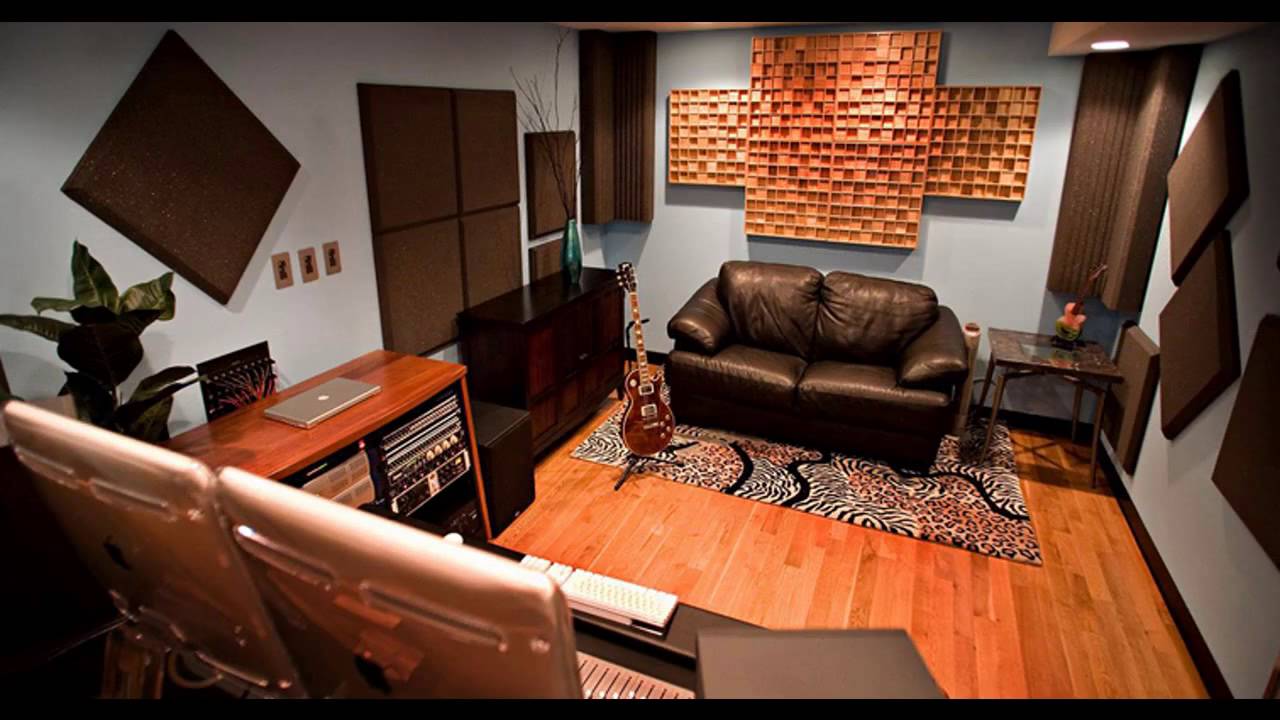This detailed image captures a studio-style music recording room with a baby blue wall backdrop. Prominent on the back wall is a display of small cork squares arranged in a cross-style pattern, accompanied by strategically placed soundproofing foam in both diamond and square patterns. 

Dominating this space, a black leather sofa stands atop a vibrant leopard and zebra print rug. In front of the sofa, a brown guitar rests on a stand. To the sofa's right, there is a brown table, while a silver Apple laptop sits on wooden stereo equipment in a cabinet to the front left-hand side of the image.

The room features additional soundproofing materials, especially in the corners, to enhance sound quality. There is also a blue shelf along the left wall, housing various records and music equipment. A potted green plant adds a touch of nature, placed on the entertainment center. Spotlights illuminate the space, highlighting the detailed and functionally arranged elements throughout this music studio.